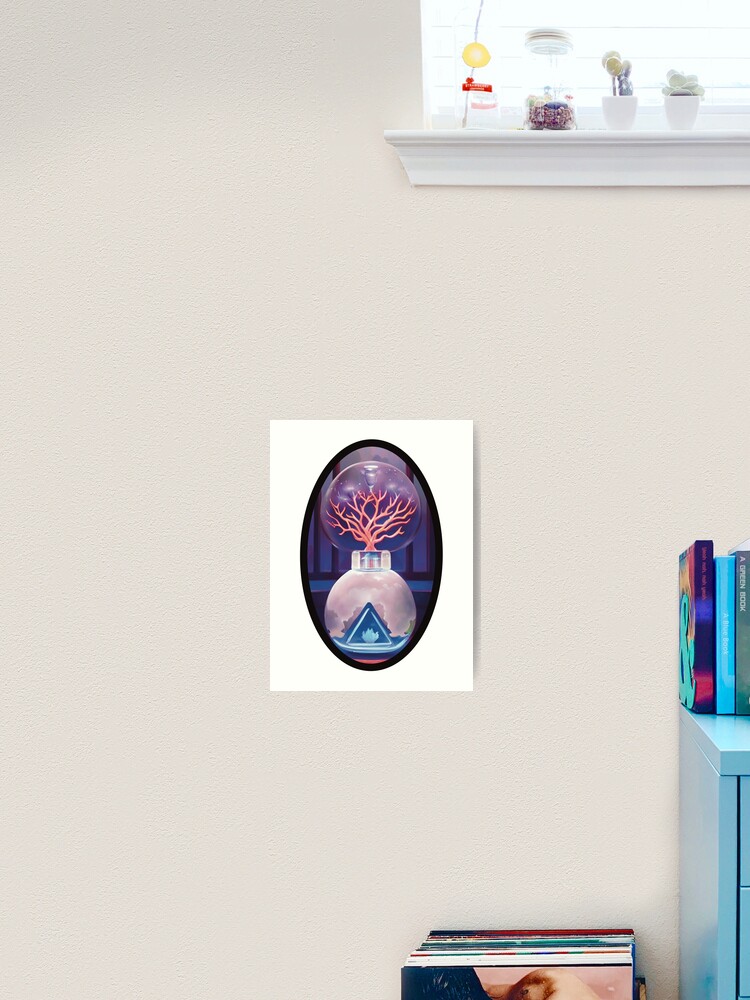The image depicts a beige-colored wall inside a room, adorned with various items and furnishings. Toward the top right corner, a white shelf, which appears to be part of a windowsill, holds a collection of knickknacks, including bottles and jars with colors predominantly in clear, white, red, and yellow, as well as two succulents in white pots. Centered on the wall is a rectangular white-framed picture that features an oval-shaped centerpiece. Inside the oval, there is an intricate depiction of reddish-pink vines or coral growing within a clear glass globe, which has a gray bottom and a small blue triangle on the side, all set against a blue and purple background. In the lower right corner, the edge of a blue cabinet is visible, with books in various colors (including purple, blue, aqua, baby blue, green, red, aqua, white, black, blue, and pink) stacked on and around it. A possible stack of LP records or a box can be seen in the lower central area, adding to the eclectic yet harmonious decor of the room.